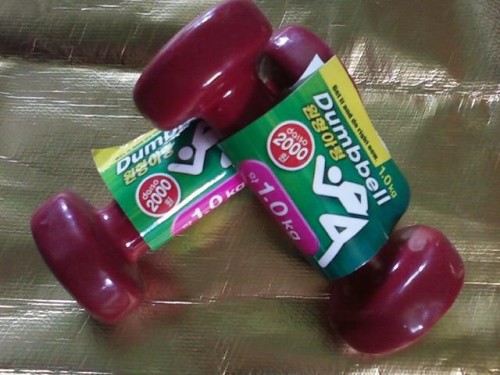This close-up image features two brand new, dark red dumbbells arranged in a crisscross fashion, with one resting on top of the other. The dumbbells are adorned with green labels that prominently display the word "dumbbell" in white text, as well as a small illustration of a person lifting weights. Additional details on the labels include yellow symbols and text in what appears to be an Asian language, possibly Chinese. A purple rectangular section on the labels clearly indicates the weight of the dumbbells as 1.0 kg. These light-weight dumbbells are likely intended for light exercises or physical therapy. They are placed on a brown surface with a textured, tarp-like, possibly plastic material that shows some wrinkles.